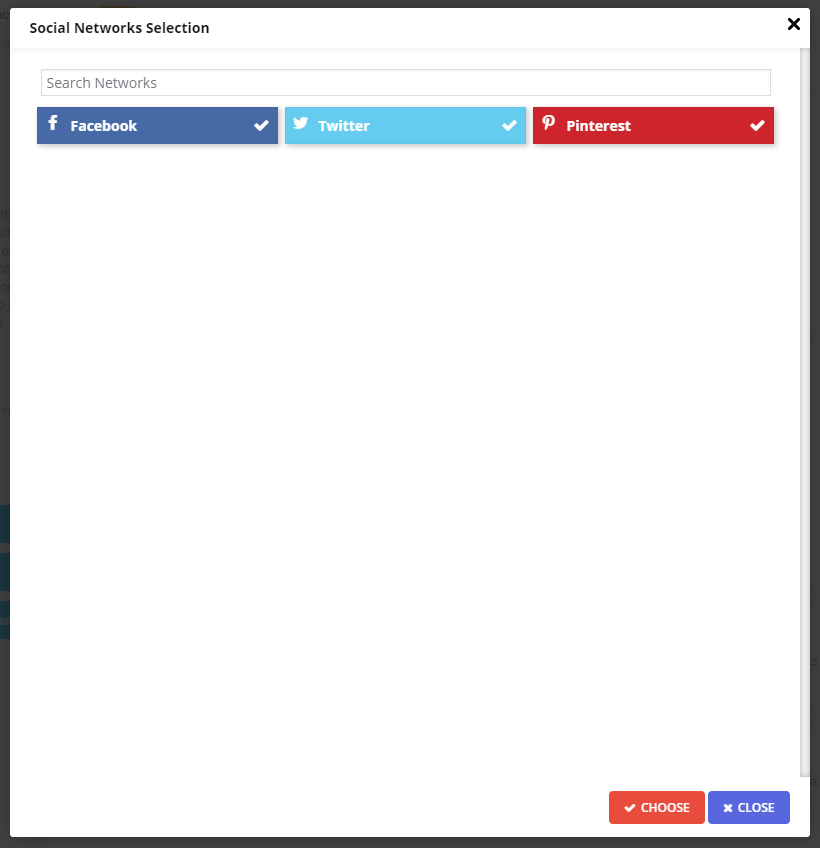The image features a predominantly white square bordered by black lines. At the top left corner, the text reads "Social Network Selection," while the top right corner displays a small 'X'. Below the header, three vertically aligned rectangles represent different social media platforms: Facebook in dark blue, Twitter in light blue, and Pinterest in red, with each platform name written in white within its respective rectangle. At the bottom right corner of the image, there are two options presented in rectangles: a red rectangle labeled "Choose" marked with a checkmark icon, and a blue rectangle labeled "Close" accompanied by an X icon. The overall design is clean and organized, directing the user towards selecting a social network or closing the selection interface.